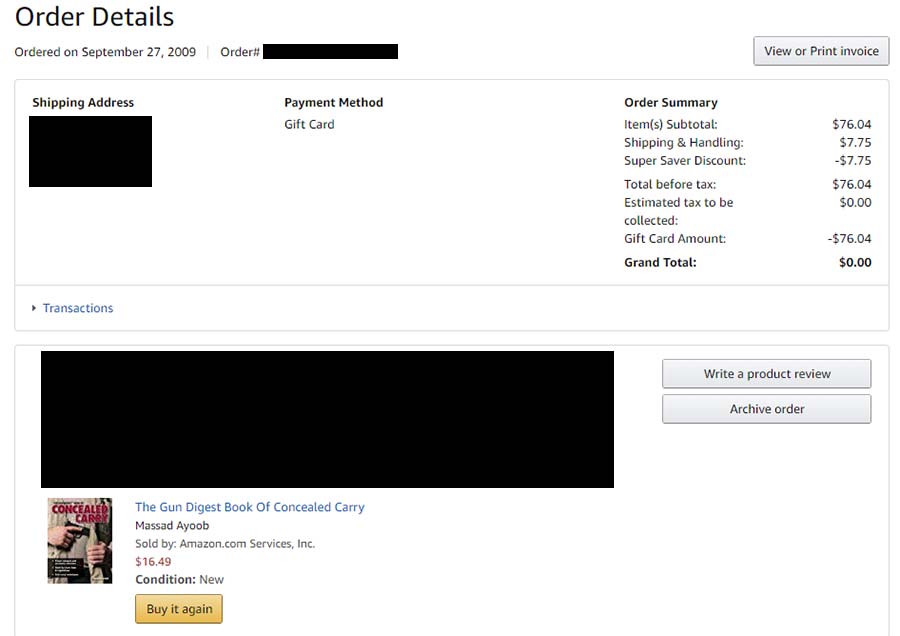The image displays an order confirmation page with various details masked for privacy. The background is white with black text. 

In the top-left corner, the heading "Order Details" is prominently displayed, followed by the subheading "Ordered on September 27, 2009." Below this, the order number is obscured with a solid black bar. In the top-right corner, there's a button labeled "View or Print Invoice."

On the left side, the label "Shipping Address" appears with the actual address covered in solid black. At the center of the image, the payment method is listed as "Gift Card."

To the right, an "Order Summary" section itemizes the costs:
- Items Subtotal: $76.04
- Shipping and Handling: $7.75
- Super Saver Discount: -$7.75
- Total Before Tax: $76.04
- Estimated Tax to be Collected: $0.00
- Gift Card Amount: -$76.04
- Current Total: $0.00

At the bottom-left of this section, the term "Transaction" is written in blue. Below, a large black box obscures additional details, but it's clear that one of the items listed is a product titled "Concealed Carry" by Mazat Ayub, sold by Amazon.com Services for $16.49 in new condition. 

To the far right, there are two gray buttons labeled "Write a Product Review" and "Archive Order," alongside a yellow button that says "Buy it Again."